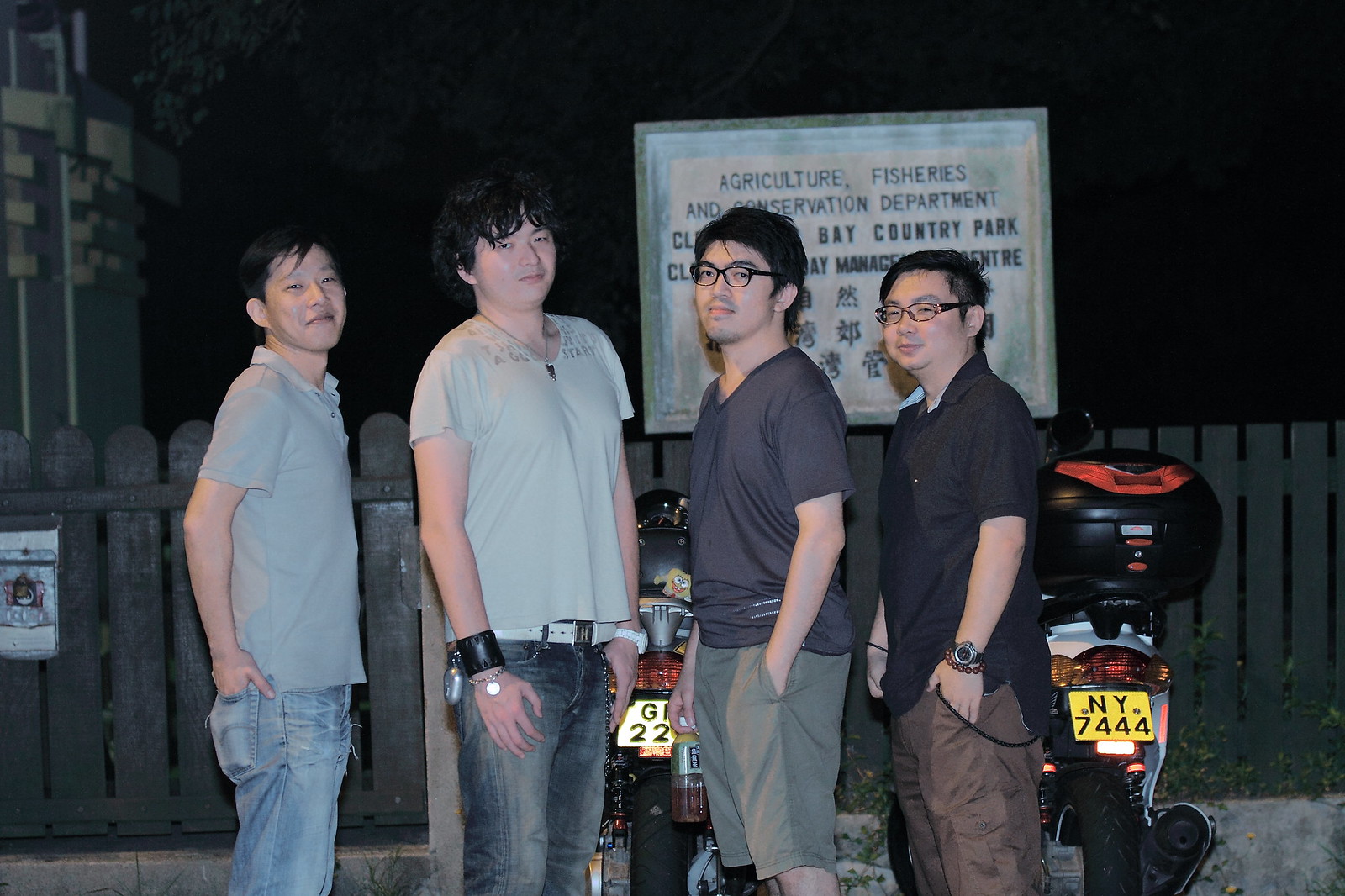The photograph captures four Asian men posing at the center of the image. From left to right, the man on the far left has short black hair, a light gray polo shirt, and blue jeans, with one hand in his back pocket. He stands in a side profile while looking directly at the camera. The next man to his right also has black hair, albeit curly and scraggly. He wears a light gray V-neck t-shirt, blue jeans, a leather bracelet, and a white watch. He, too, faces the camera directly. The third man, positioned at the center right, sports short black hair and black-framed glasses. Dressed in a dark gray V-neck t-shirt and dark green shorts, he stands in a side profile, with one hand in his pocket. The man on the far right has short black hair, black-framed glasses, a black polo shirt, a black watch, a small red bracelet, and dark brown pants. He gazes slightly off to the left of the camera.

In the background, behind the men, there are visible motorcycles or scooters, primarily black, one of which has a yellow license plate with the number "NY 7444." Another partially obscured license plate shows the characters "G22." Also, a sign reads "Agriculture, Fisheries, and Conservation Department," although it is partly hidden by the men. The scene appears to be set at night, with a dark backdrop featuring a wooden fence that reaches the men’s waist height, a few tree branches at the center top, and a cropped building visible at the very top left of the image.